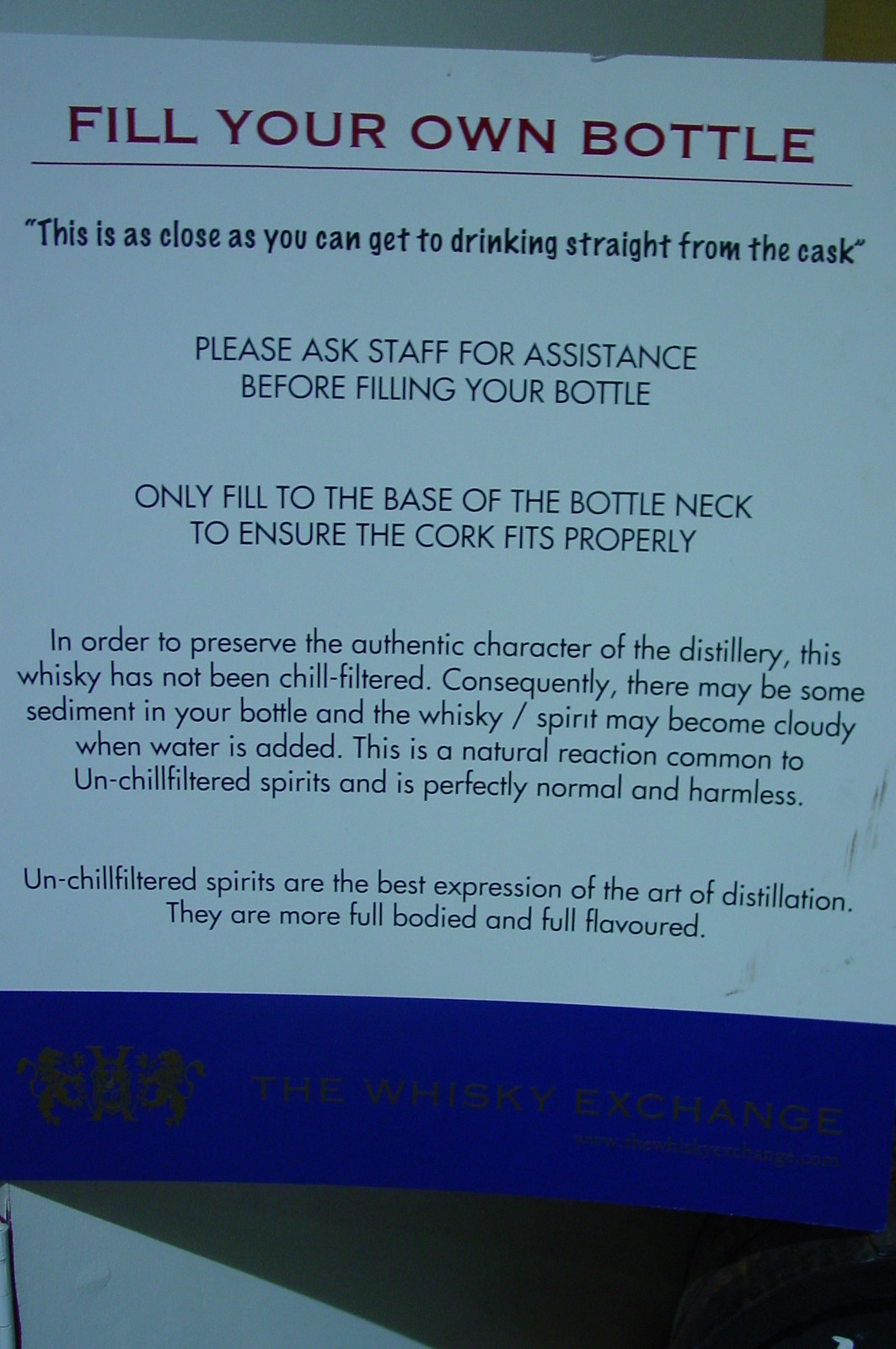The image shows a sign with detailed instructions for filling your own bottle with whiskey. The sign, set against a somewhat light blue-tinted background with a blue border, features bold, red, capitalized text at the top stating "FILL YOUR OWN BOTTLE," underlined by a red line. Below, in dark blue or black text, it reads: "This is as close as you can get to drinking straight from the cask." Further instructions advise asking staff for assistance before filling your bottle and gently filling to the base of the neck to ensure the cork fits properly. Additional notes explain that to preserve the authentic character of the distillery, the whiskey has not been chill filtered, which may result in some sediment in the bottle and cloudiness when water is added. This reaction is natural and harmless, a testament to un-chill filtered spirits' more full-bodied and full-flavored nature, highlighting their superior expression of the art of distillation. At the bottom of the sign, over a blue background, is the text: "The Whiskey Exchange."